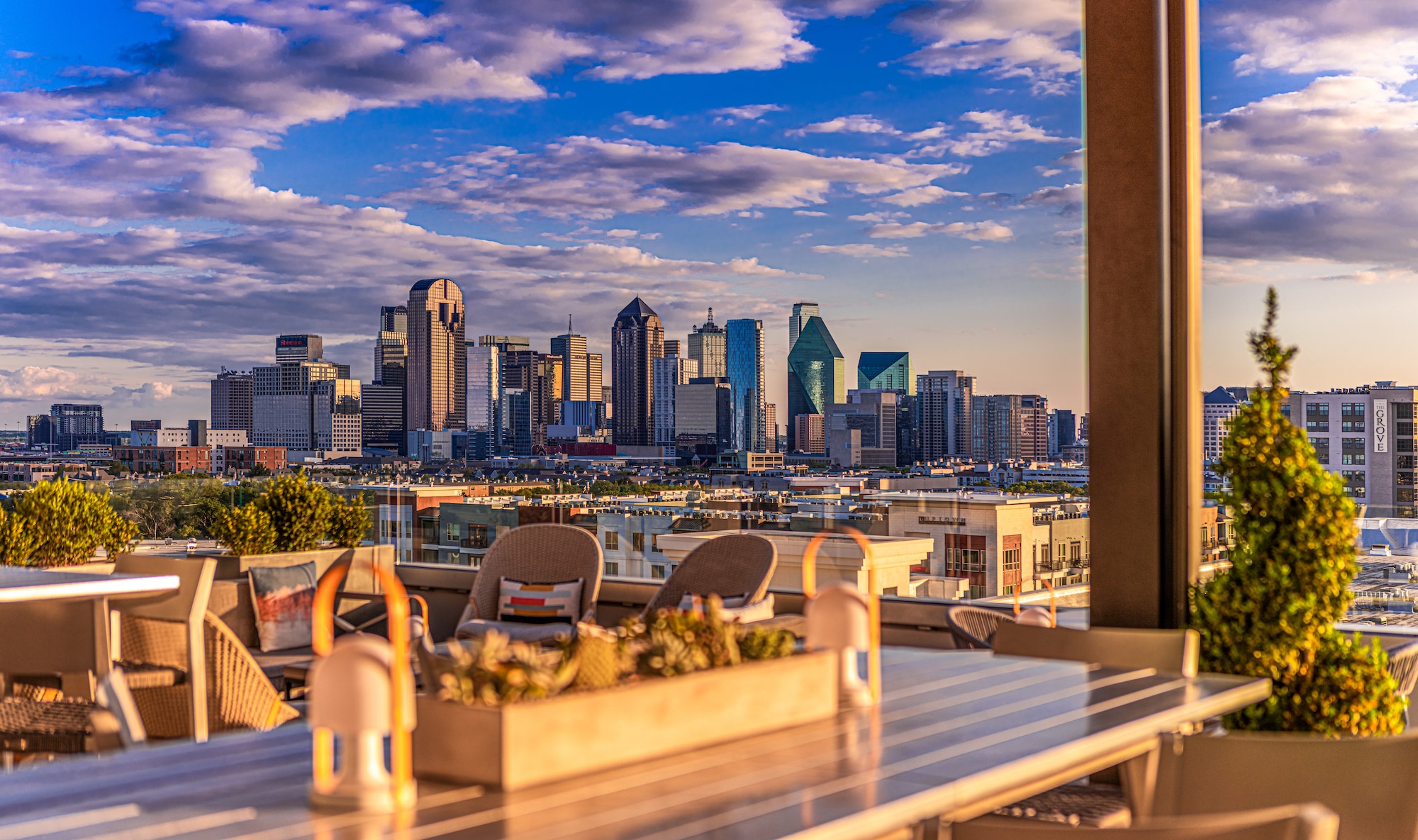The photograph captures a picturesque and well-maintained courtyard, likely part of a hotel or upscale residential building, adorned with neatly arranged outdoor park-bench-style tables. Dominating the foreground is a prominent table extending from the bottom edge of the image, complemented by another situated about six feet to the left. A white potted plant is conspicuous on the right side of the frame, hinting at an outdoor pergola or roofing structure overhead, as evidenced by a vertical column or post emerging from the right edge. 

The background transitions into an impressive city skyline, showcasing a blend of towering skyscrapers with varied architectural designs—some are tall and square, others dome-shaped, and one notably round with reflective glass. The skyline is framed by a neighborhood of apartment buildings and city blocks below the deck. Overhead, the sky presents a dynamic palette of blue interspersed with gray clouds, adding depth and liveliness to the scene. Additional potted plants dot the lower left side of the photo, enriching the inviting ambiance of this rooftop-like balcony area.